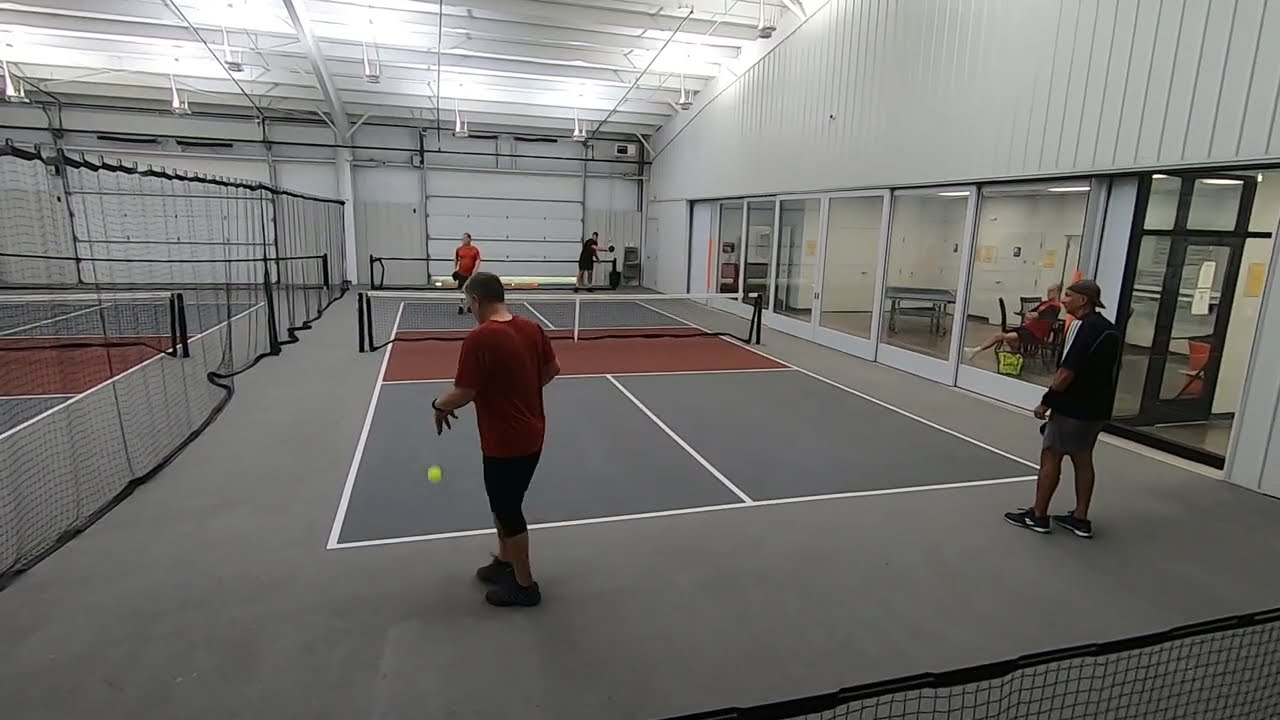The image depicts an indoor tennis court scene framed by a steel structure with multiple beams and overhead lights. The court surface is a mix of gray and tan hues, highlighted with white lines and anchored by a darker red stripe where the net stretches across. In this game, four men are in the middle of a match, prepared for the serve. On the right side, a man in a black shirt, gray shorts, and black shoes stands ready, while beside him, a man with a backward baseball cap, dressed in a red shirt and black shorts, is about to serve a yellow tennis ball with his left-hand wrist adorned in a black watch. Opposite them on the left are two more players: one in a red shirt with black shorts and shoes and the other in a black shirt, black shorts, and white shoes. The tennis court is enclosed by a black wire fence that separates it from another adjacent court. To the right, there is a room with white steel panels and glass doors, where a lone man sits on a chair over a yellow container, viewing the match.